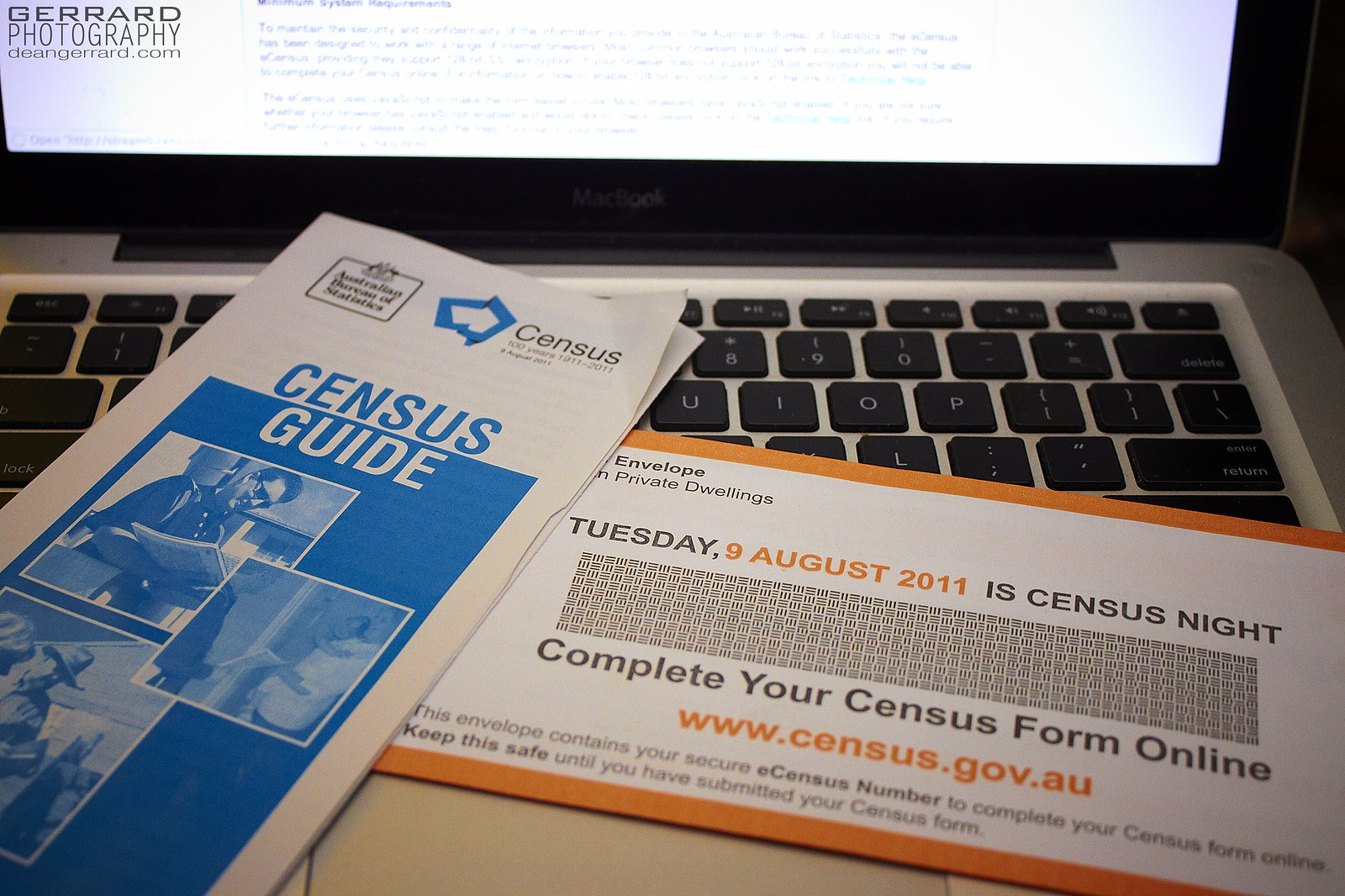The image is a wide, rectangular photograph capturing a portion of a silver MacBook laptop, specifically the keyboard and a small section of the screen at the top. The keyboard features black square keys with white lettering. Placed diagonally from the bottom right to the top left of the keyboard is a white envelope with an orange border. The envelope reads in a combination of black and orange text: "Tuesday 9 August 2011 is Census Night, complete your census form online, www.census.gov.au." The envelope is partially overlapped by a brochure to the left, titled "Census Guide." The brochure has a white background and features a blue logo at the top, accompanied by the word "census" in black text. The body of the brochure incorporates a sequence of three blue-tinted photos with white borders, depicting individuals engaged in various activities. One photo shows a man looking at a book, another shows a man speaking to someone at a doorway, and the last shows a man in a cowboy hat, though the rest of this photo is mostly cropped out. Also visible at the top left of the image is a faint watermark that reads, "Girard Photography www.deangirard.com" in black text. The MacBook logo can be seen in a gray font with a black background at the top center of the image, adding to the detailed composition.